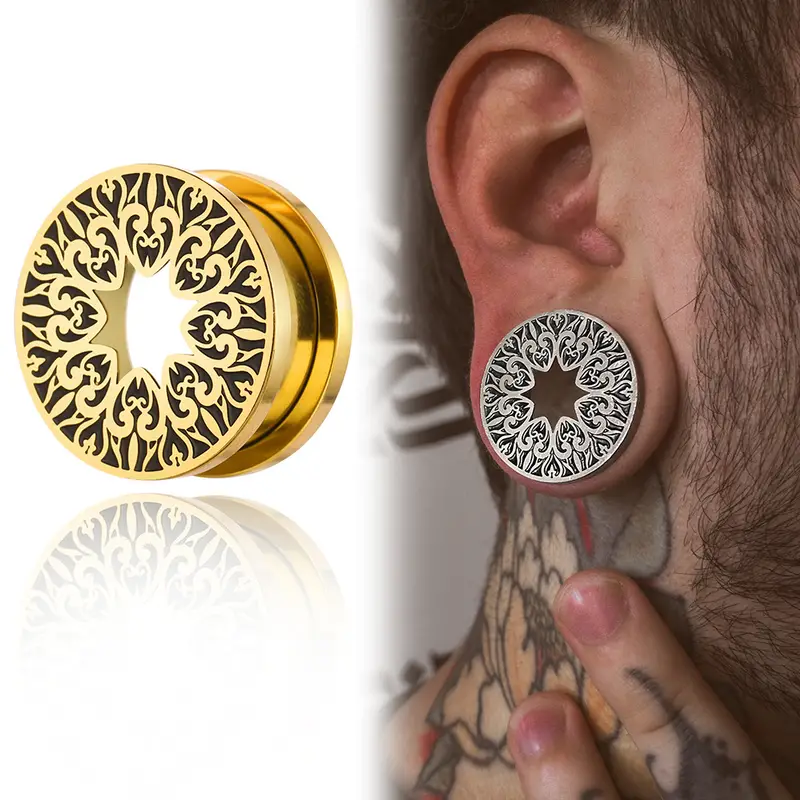The image showcases a detailed close-up of a man's ear, adorned with an intricate silver ear gauge that prominently displays an eight-pointed star design. The man's neck and fingers are heavily tattooed, and his scruffy beard is visible. His fingernails appear to be painted a pale pink hue. The right side of the image features his tattooed hand gently resting on his neck. Additionally, there is a zoomed-in view of the same ear gauge, but in a gold version, on the left side of the image. This ear gauge, about two inches in diameter, features heart shapes around the central star and is mirrored below to emphasize its detailed design.